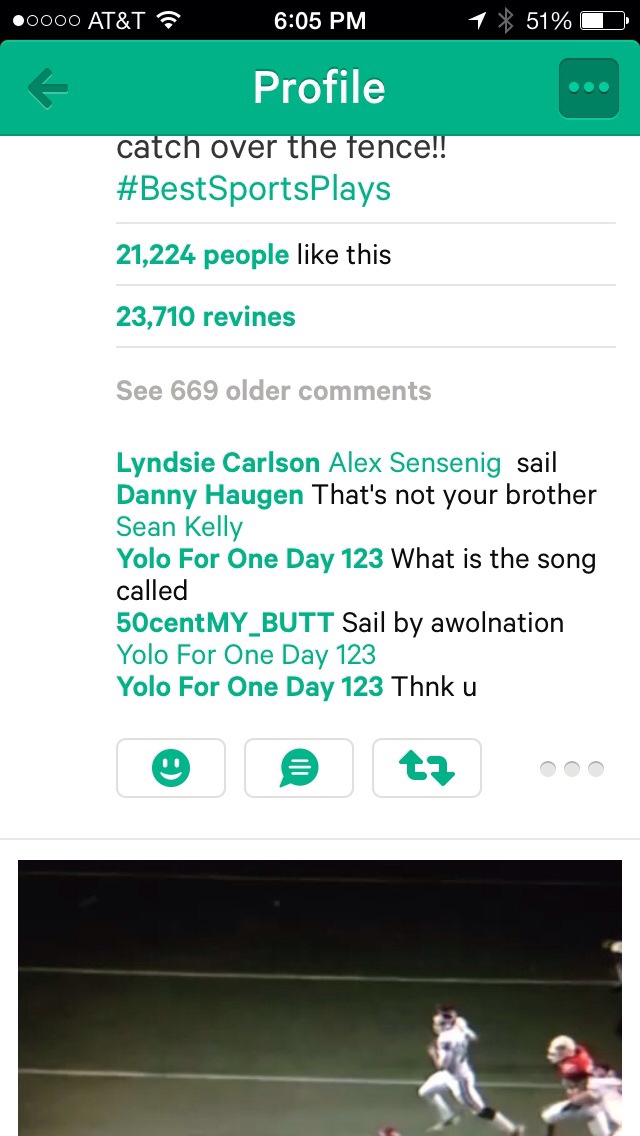The image captures a detailed screenshot from a phone screen. At the top of the screen, a thin black strip features the AT&T carrier name, along with a Wi-Fi symbol, the time displayed as 6:05 p.m. in white text, and various icons including a Bluetooth symbol, a battery life indicator at 51%, and other status icons. Directly below, a green rectangular bar is seen with a left-pointing arrow on the left, the word "Profile" centered in white, and additional icons on the right.

Following this, the main content of the screen includes a prominent post titled "catch over the fence" written in black letters, with a subheading "#best sports plays." The post shows that it has been liked by over 21,000 people and revined multiple times. Below the post, there's an invitation to see "69 older comments," after which follows a series of comments from five or six people, each name displayed in green with their comments in black text. Towards the bottom of the screen are four reaction icons enabling users to like, repost, or message.

Finally, at the very bottom of the screen is a color photograph in landscape orientation depicting a night scene on a football field. The photo shows two football players on the right; one is running to the left with the ball in his right arm, wearing a black helmet, while another player in a different uniform gives chase. The picture is somewhat cut off on the right, but the action is clear and dynamic, emphasizing the sports theme of the post.